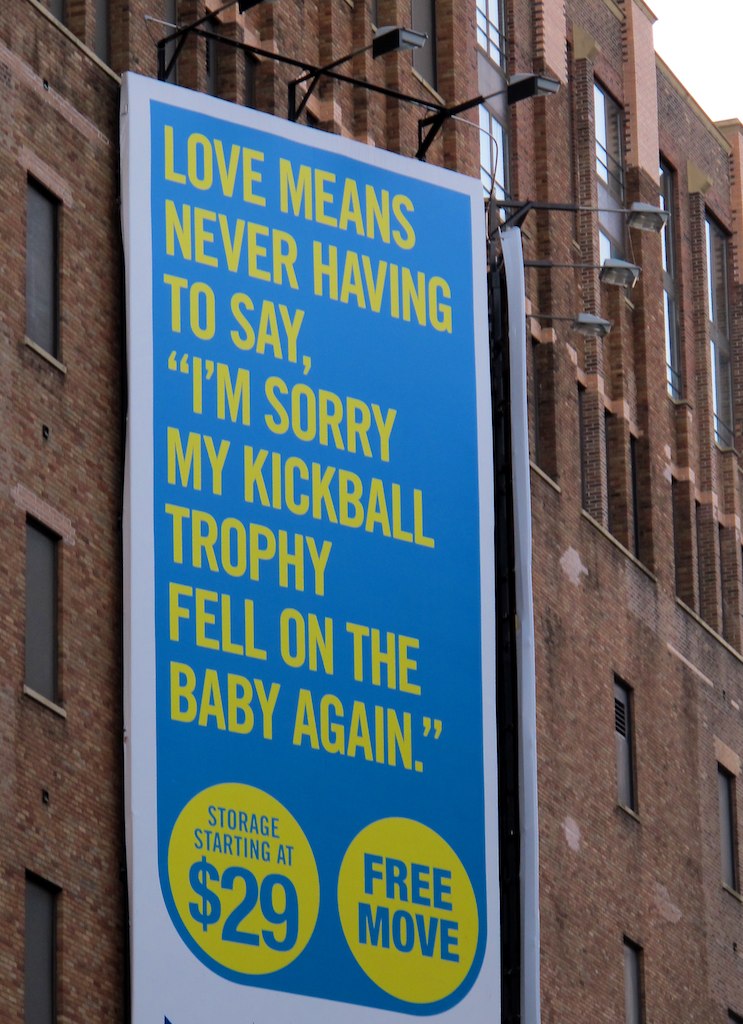The photograph, taken in color and portrait orientation, showcases a large outdoor advertisement affixed to the façade of an old brick building, likely an apartment or warehouse building situated in a city. The sign, set against a white-bordered billboard, features a blue background with bold, uppercase yellow text that reads, "LOVE MEANS NEVER HAVING TO SAY I'M SORRY MY KICKBALL TROPHY FELL ON THE BABY AGAIN." Below this text are two yellow circles with blue writing that state "Storage starting at $29" and "Free move." The advertisement spans several stories of the building, which is characterized by its closely connected, old brown brick structure with numerous windows. The image also captures gray and black streetlights and beams, emphasizing the urban setting. The photograph was taken during the daytime, providing a clear and detailed view of the scene.